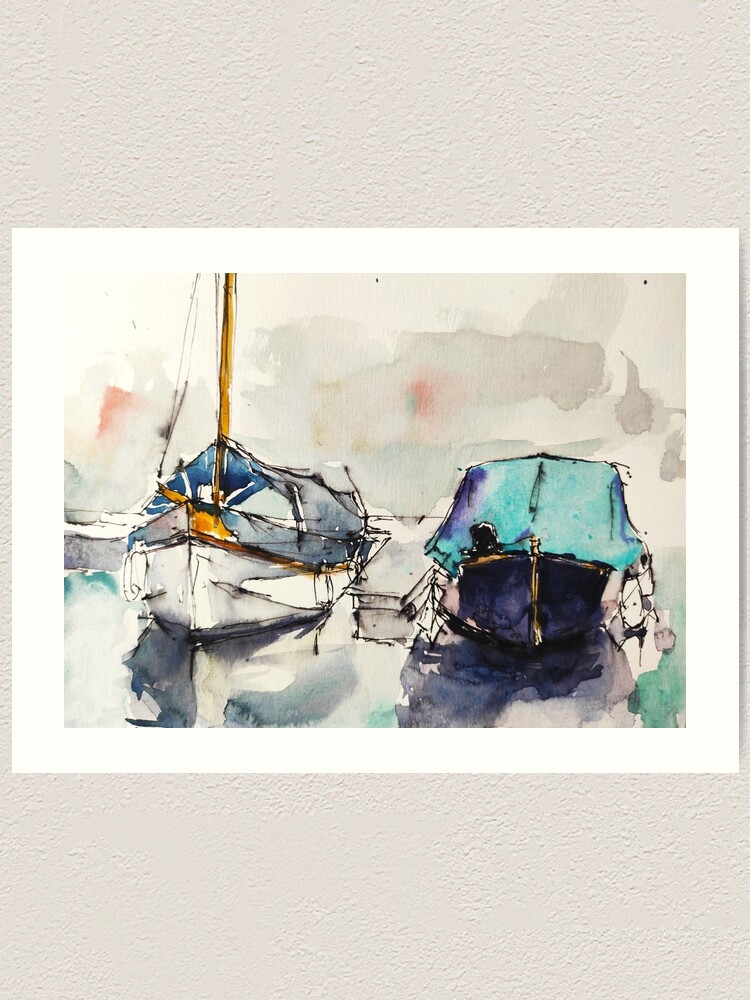The image is a digital photograph of a framed, watercolor sketch painting. The painting is mounted against a light beige, pebbled wall, and is surrounded by a white border. The scene depicts two docked boats. The boat on the left is white with a light blue canopy, featuring a tall, tan (or yellow) mast. The boat on the right, which is a speedboat, is dark blue, almost black, with a baby blue (or turquoise) colored canvas tarp protecting it. Both boats have buoys hanging off their sides to protect them from damage. In the right-hand corner, there appears to be a figure walking on the dock towards the boats. The sky in the painting is rendered in light gray tones, giving a hurried, artistic impression through the less detailed watercolor edges. The overall composition uses colors such as gray, white, blue, and teal, providing a soft and serene maritime scene.